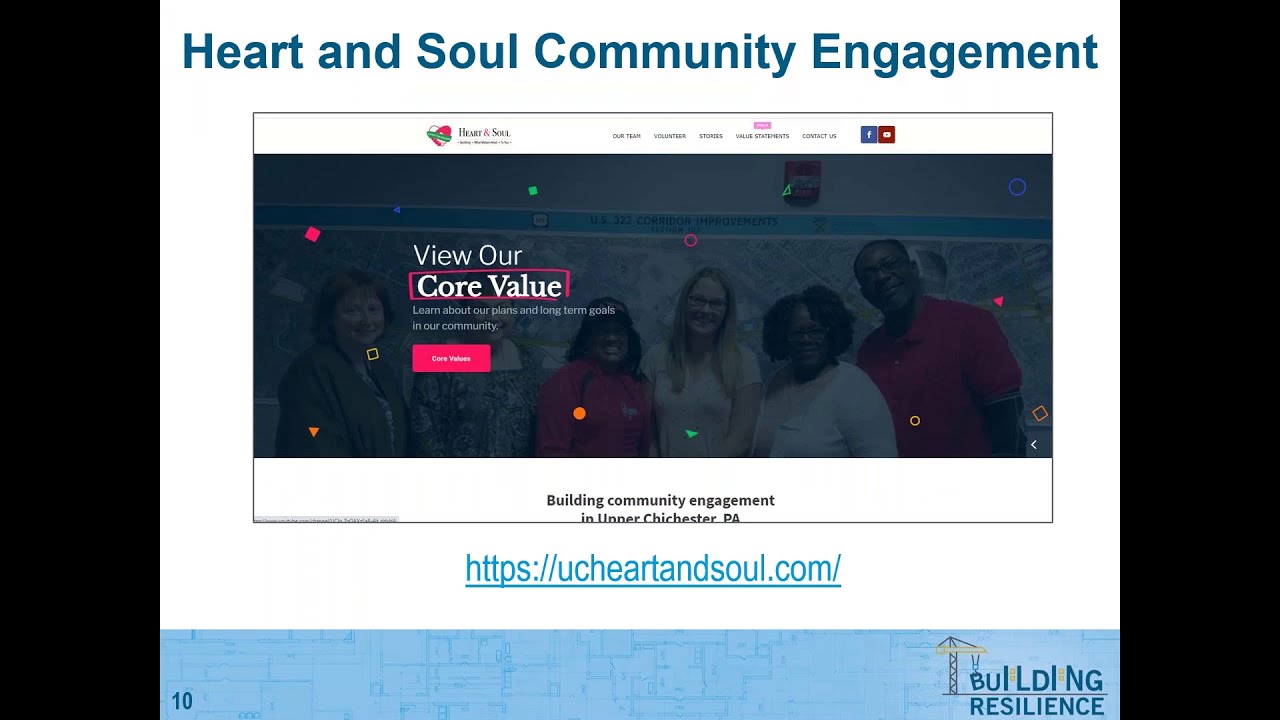This horizontal rectangular image is a screenshot of a web page viewed on a computer or cell phone screen. The image is framed with vertical black bars on both the left and the right sides. The primary background within the frame is white. At the top of the image, a headline in upper and lowercase dark blue letters reads "Heart and Soul Community Engagement". Below this headline is a darkened, almost indiscernible photograph of a group of people in a professional setting, standing side-by-side. Overlaid on this photograph is the text "View Our Core Value" in white, accompanied by a red rectangular button labeled "Core Values". Additional text beside the photo reads, "Learn About Our Plans and Long-Term Goals in Our Community".

The webpage screenshot also features navigational and social media buttons along the top banner and a small logo displaying "Heart and Soul" with a red and white heart logo wrapped in a green banner. Beneath the photograph, there's a caption that states "Building Community Engagement in Upper Chichester, Pennsylvania" and a URL in medium blue, https://ucheartandsoul.com/. At the very bottom of the image is a blue horizontal line containing the "Building Resilience" logo in the bottom right corner; this logo showcases black, playful handwritten-style lettering of various sizes.